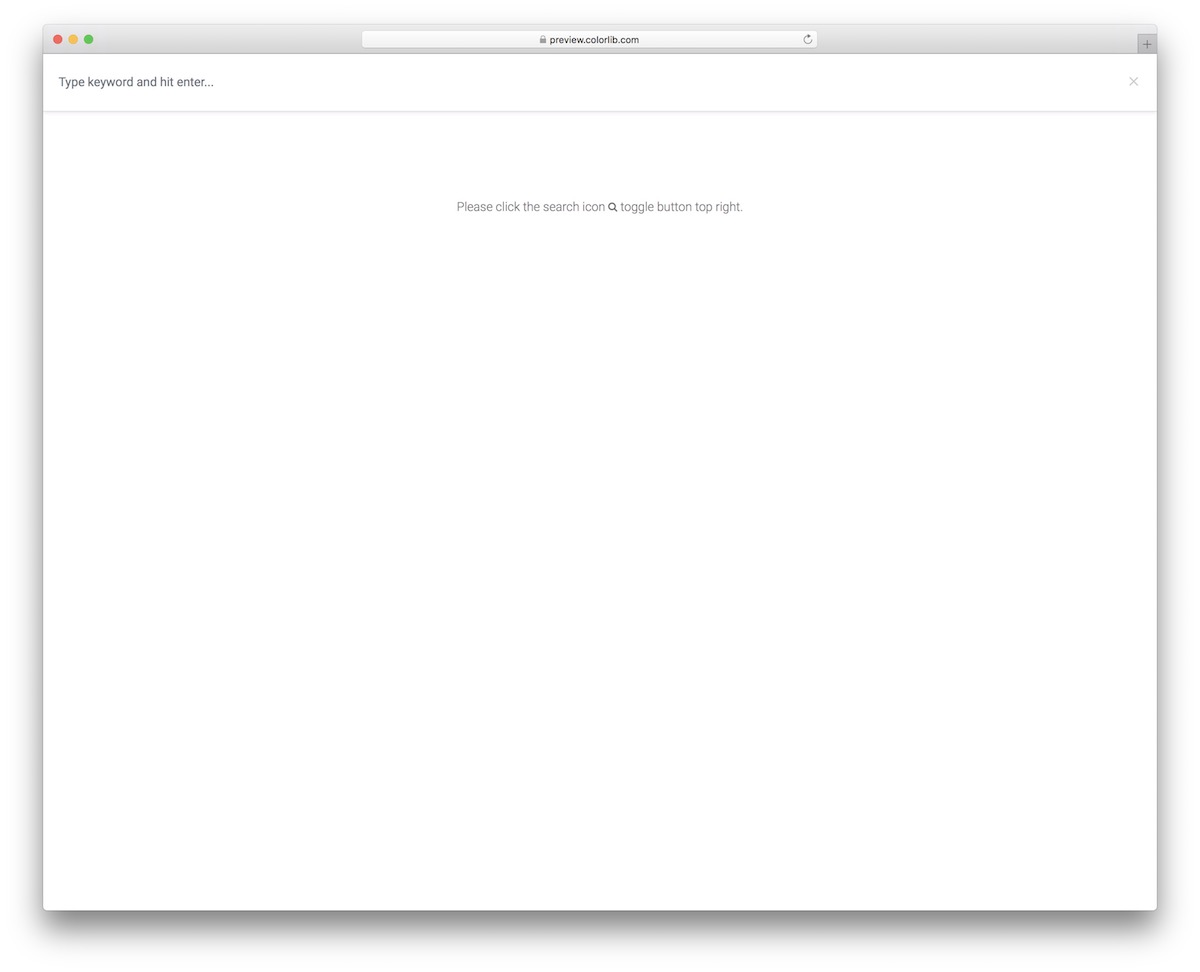The image depicts a web browser window with its main display area currently empty and presenting a white background. Dominating the top section of the browser is a gray bar, which spans the entire width from left to right and features a subtle gradient, transitioning from a lighter tone at the top to a slightly darker one at the bottom.

On the left side of this gray top bar are three colored circles arranged horizontally – a red circle, a yellow circle, and a green circle, which are typically used to represent window control buttons (close, minimize, and maximize, respectively).

Situated at the center of the gray bar is the browser's address bar. Inside the address bar, there is black text displaying "preview.colorlib.com," flanked on the left by a padlock icon, indicating a secure connection, and on the right by a refresh symbol, suggesting the ability to reload the page. Towards the far right of the top gray bar is a small "X" icon used for closing the browser window or tab.